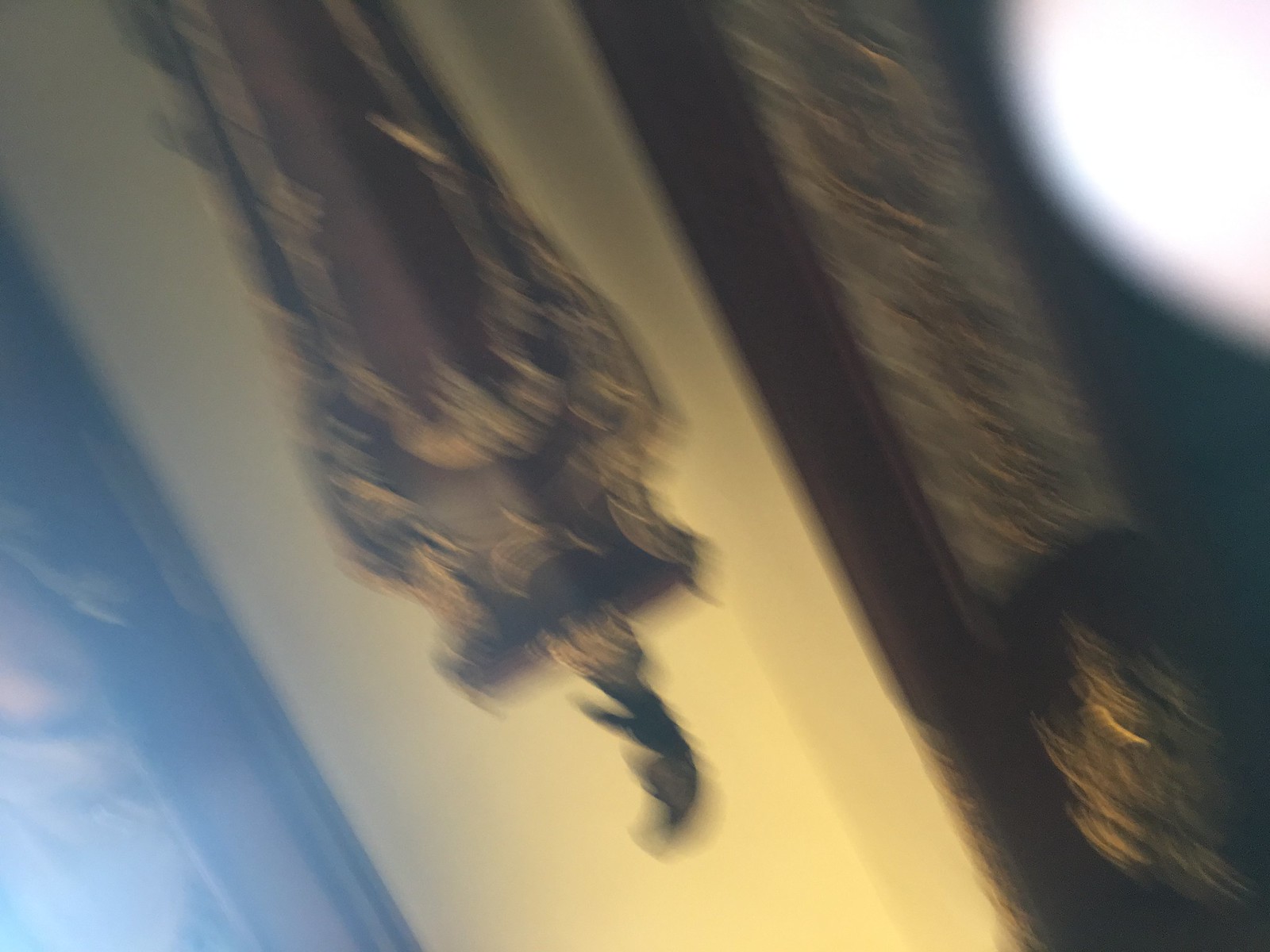The image is a very blurry and out-of-focus photograph, taken at a slight angle. In the upper right corner, a bright, white semicircle area suggests some light source. Adjacent to this, a rectangle with a black outline and golden, crumpled interior material is visible, resembling a foil. 

Dominating the center is a beige background with an off-white wall, featuring a black, mirror-shaped item adorned with yellow or gold decorations and a fin-like extension at the bottom. The bottom left corner is notably lighter, possibly due to an area of light. To the right, dark areas hint at wooden elements, possibly a door frame. The unclear, elongated black shape with a decorative fin seems to be a wall-hung item, perhaps evoking comparisons to a weapon like a sword from Soul Calibur.